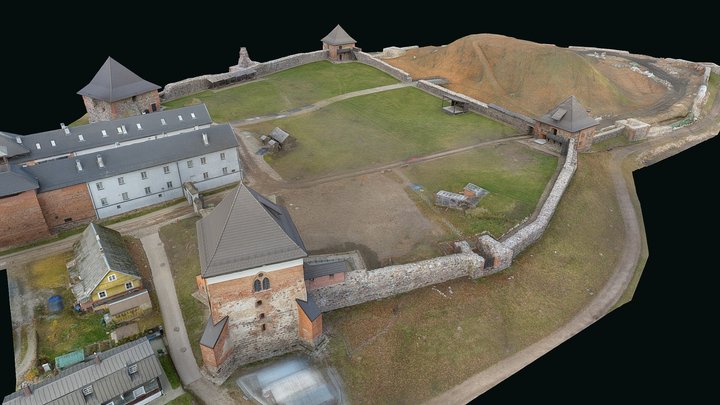An aerial photograph depicts an old-time fort situated on a small island, entirely surrounded by water. The fort is enclosed by robust rock walls with little guard houses strategically placed at the corners. Within the fort's walls, there are approximately eight buildings of various architectural styles, including some with slanted and hip roof designs. The structures vary in age; some appear to be several hundred years old, while others look newer or refurbished. These buildings include two larger ones, possibly used to house people, and a smaller one that resembles a farmhouse. One of the buildings is notably yellow. The scene is rich with colors like brown, green, and rust, highlighting open fields with green grass both inside and outside the fort's walls. In the background, there's a hillside with a path leading to the top. The entire area is surrounded by deep, clear water, and the photograph has a blacked-out background, with no visible text or people present in the image.